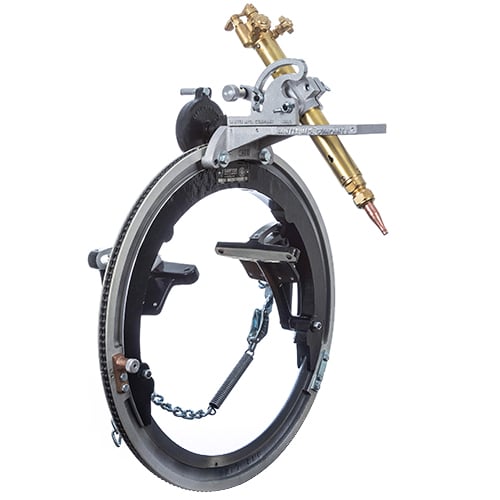The image depicts a Sawyer quick saddle beveling machine against a white transparent background. The primary structure features a large circular metal ring, silver in color, with an interior circle that is black. Around the perimeter of the outer ring is what appears to be a gear chain. Central to the machine, a chain with a spring connects various metal components inside the ring. Two clamps within this circle hold in place a golden instrument resembling a pen, which projects outward from the top of the circle. Adjacent to this, a metal piece stretches across the circle. On the left side, there's a crank handle likely used for adjustments. Despite some illegible writing on the top, the overall design showcases the intricate and precision-crafted nature of this beveling machine.